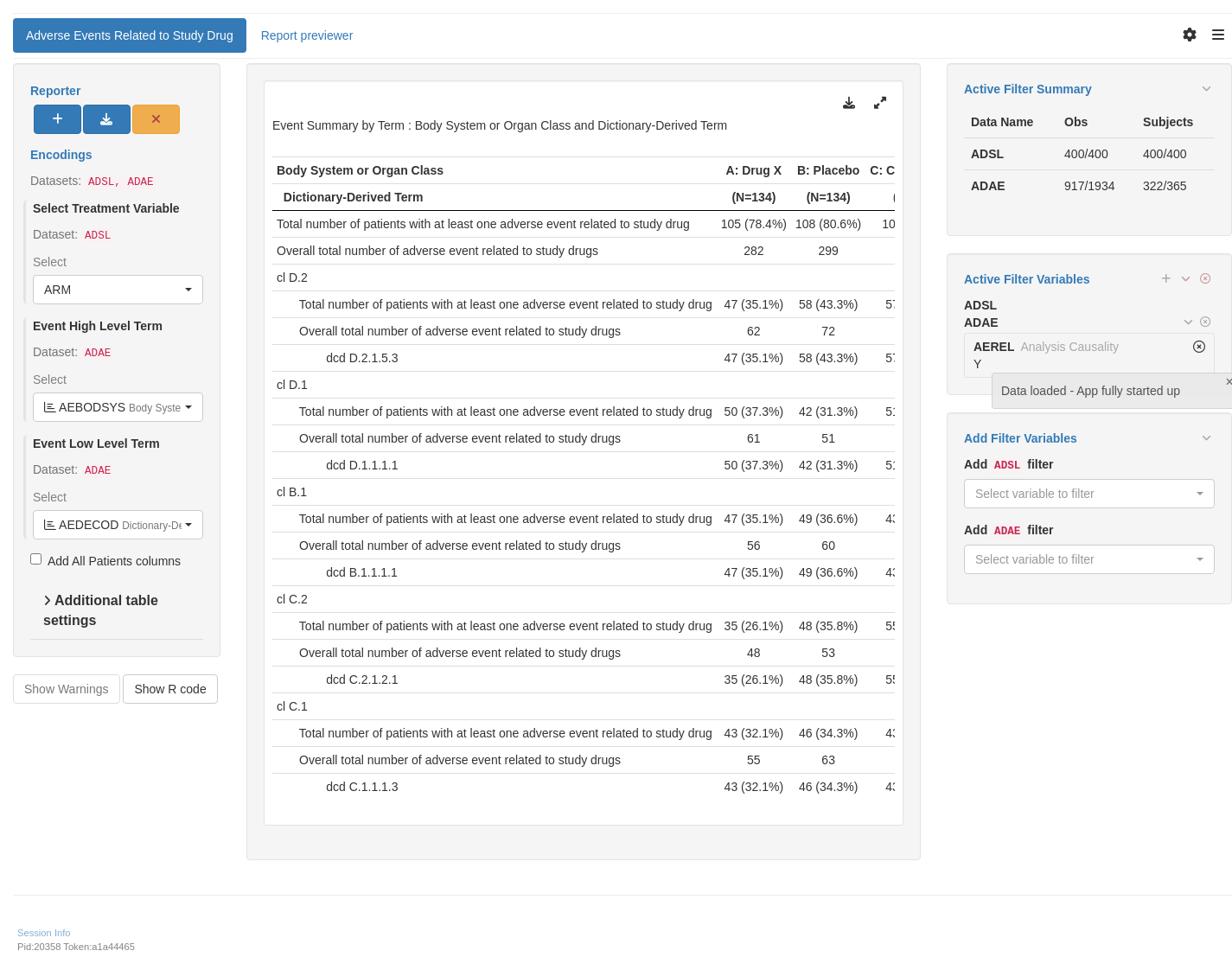This is a detailed and cleaned-up caption for the described screenshot:

---

The image is a screenshot of a website or application interface, featuring a clean white background with multiple information-filled sections. On the left side of the screen, there is a sidebar titled "Reporter." To the right, three distinct boxes are vertically aligned: "Active Filter Summary," "Active Filter Variables," and "Add Filter Variables," each with a light gray background and titles in blue text.

Dominating the center of the page is a large section filled with lines of text against a light gray background. Nestled within this is a white rectangle with the heading in gray text at the top left: "Event Summary by Term, Body System, or Organ Class and Dictionary Derived Term." At the top right of this rectangle are black icons for download and full-screen functionalities.

Beneath this, a thin light gray line separates it from bold, left-justified text reading: "Body System or Organ Class." On the right, after some spacing, are columns labeled "A, Drug X, B, Placebo, C, Calm," though the rest of the column titles are cut off by the frame. Another thin gray line further separates this from the subsequent slightly indented line labeled "Dictionary Derived Term." Underneath each "A, B, and C" column title, there are entries in parentheses: "(n=134), (n=134), (n=1)," though the remaining text is cut off.

Following this, additional lines of information appear, presented in gray text against the white background.

---